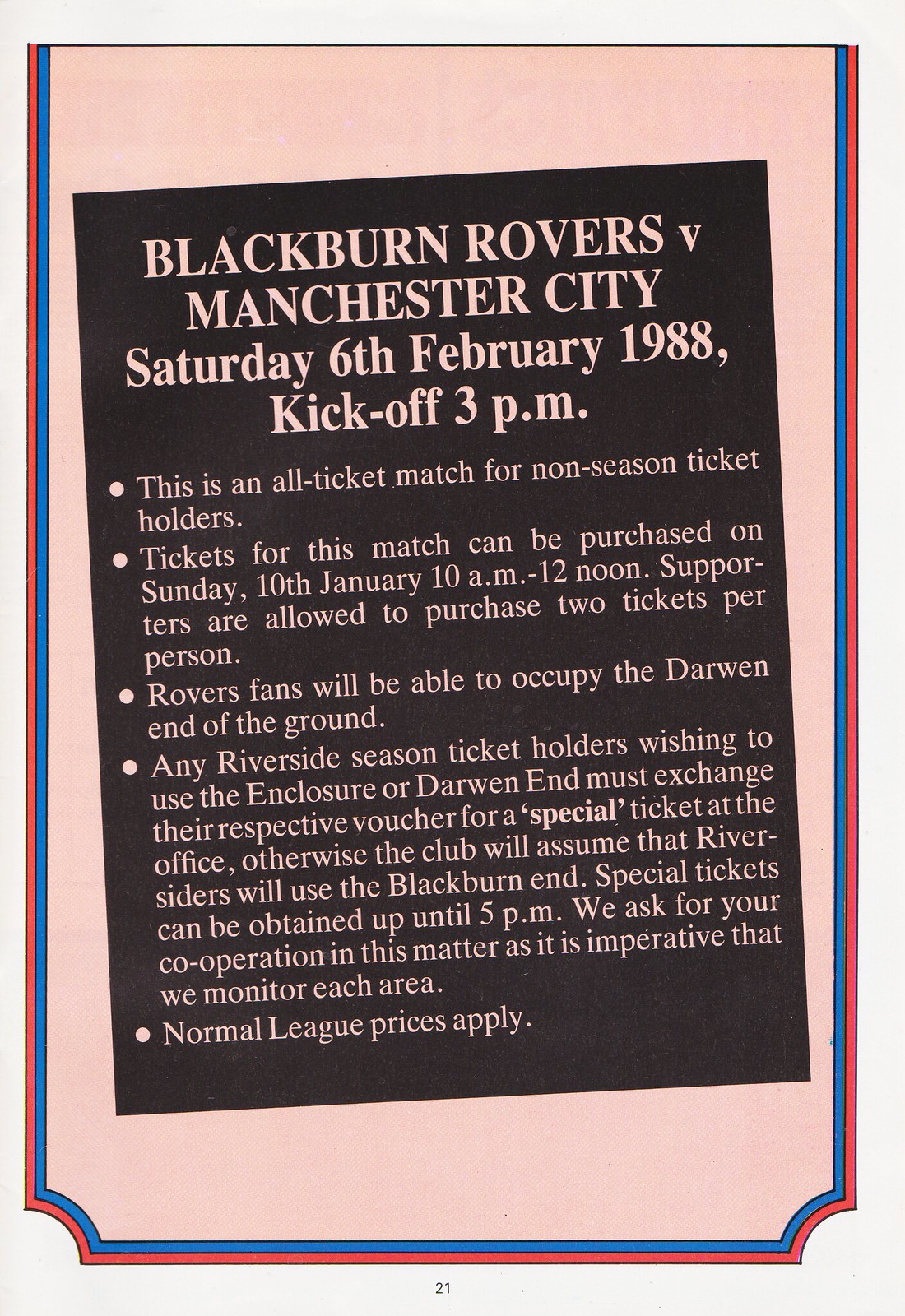The image prominently features a ticket for a UK football match between Blackburn Rovers and Manchester City, scheduled for Saturday, 6 February 1988, with a kickoff at 3 pm. The background of the ticket is primarily pink, bordered by narrow blue and pink stripes on the edges. In the center, there's a large, slightly offset black rectangle with detailed text in a pale pink hue.

The ticket indicates it’s an all-ticket match specifically for non-season ticket holders, with tickets available for purchase on Sunday, 10 January from 10 am to 12 noon. Each supporter is allowed to purchase up to two tickets per person. Rovers fans will be designated to occupy the Darwin end of the ground. Riverside season ticket holders who prefer to use the enclosure or Darwin end must exchange their vouchers for a special ticket at the office. Otherwise, it is assumed they will use the Blackburn end. Special tickets are available until 5 pm, emphasizing the need for cooperation to monitor each area effectively. Normal league prices apply.

Additional information is provided beneath the main text on the ticket, supporting the need for clear and organized seating arrangements for the match.